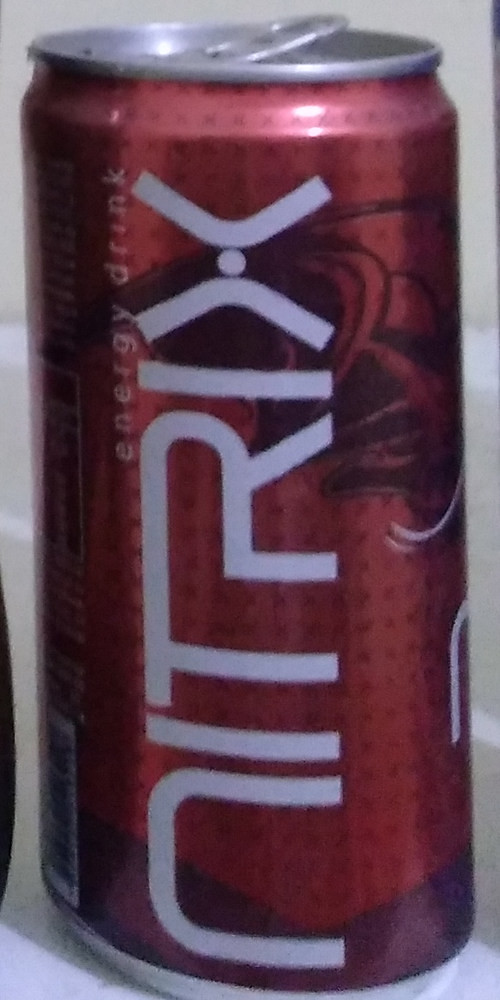Image Description: The image captures a metallic red can prominently positioned against a grey background, likely set on a countertop. The can is adorned with black speckles and features an intricate black design in the background. At its center, bold text spells "Nitrix" with the letters "T" and "R" stylized to share a conjoined top, and a distinct dot positioned in the middle of the "X". Below the brand name, the label indicates it is an "Energy Drink". Although the nutrition label is partially visible on the side, the text is obscured and unreadable. A subtle purple band encircles the bottom edge of the can. The top of the can appears slightly tampered with, where the pop-top has been lifted minimally but not fully opened.